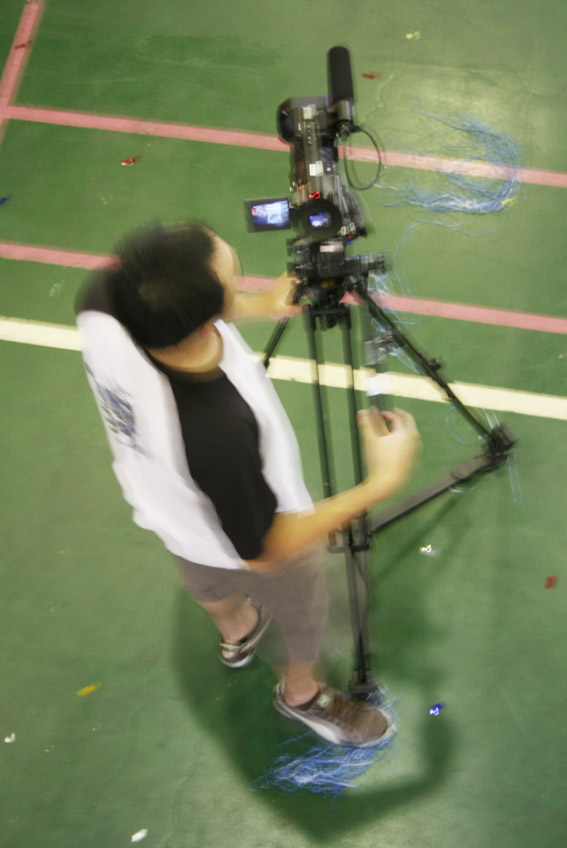This is an aerial shot taken from a high vantage point, possibly from the stands, showcasing a man operating an advanced video camera setup. The scene appears to be in an interior space with a concrete floor marred with scuffs, marks, and stains. The floor is demarcated with pink and white lines, suggesting it could be an indoor gymnasium or a stage with areas blocked off, adding to the ambiguity of whether it’s a performance or a sporting event being filmed. The man, with black hair, is dressed in a white shirt with black sleeves, khaki shorts, and brown sneakers. He stands next to a professional-grade camera mounted on a black tripod, complete with a foam-covered microphone and an open display screen. The camera is directed forward as if capturing someone or something in front of it. Despite the blurry and artifact-ridden quality of the image, the detailed setup hints at a significant filming effort, possibly a performance or an interview, on what seems to be a green surface with distinct markings.